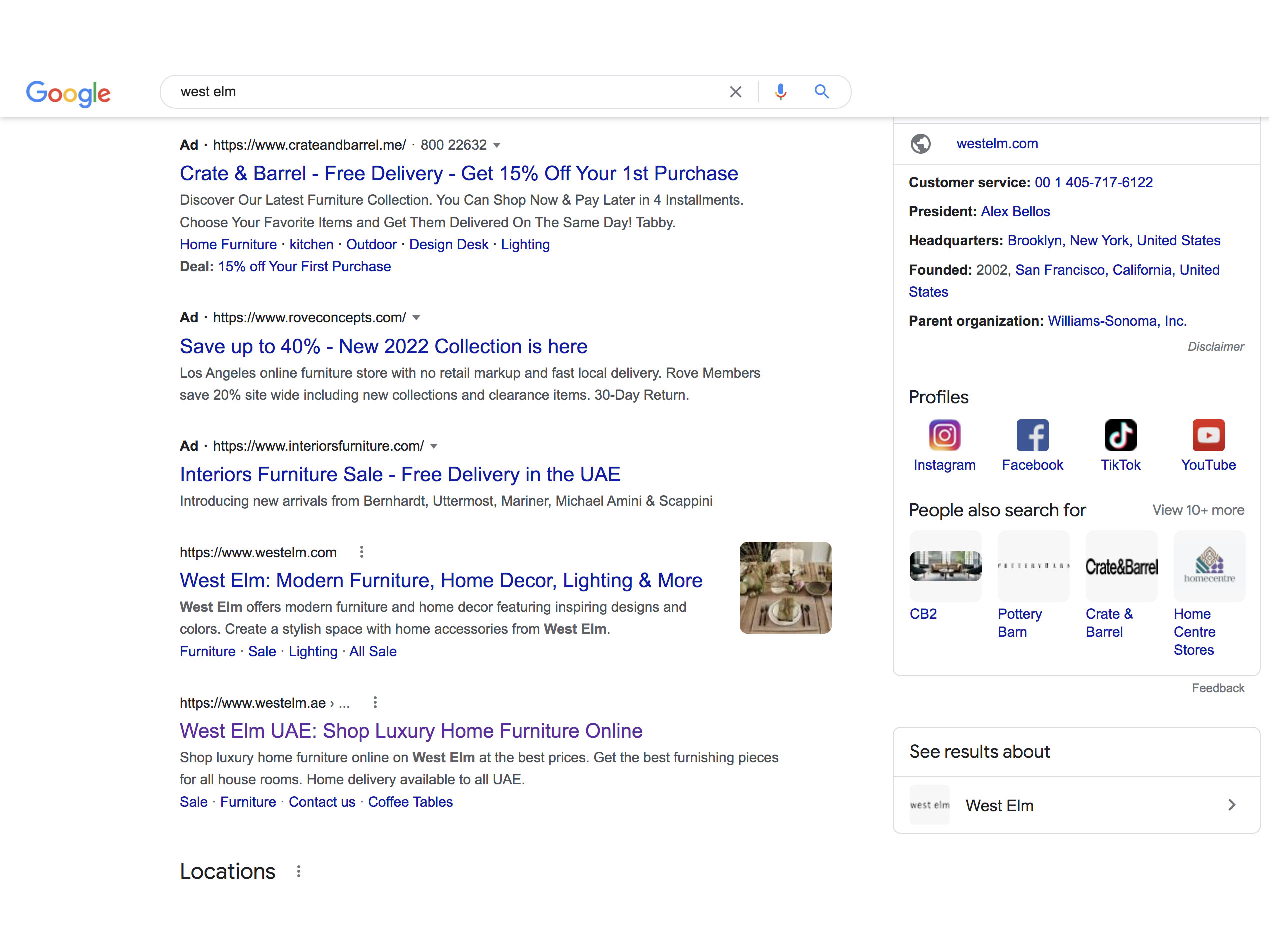This image is a screenshot of Google search results. At the top of the screenshot, there is a white header background featuring the Google logo on the left side. To the right of the logo is a search bar with a white background and a thin light grey outline. The search bar is rounded on both ends and contains the black, left-justified text "West Elm." On the far right of the search bar, there are several icons in sequence: a grey "X," a thin vertical grey line, a blue and red microphone icon, and a blue magnifying glass icon.

Below the header, the body of the page has a faint light grey shadow and a white background. The listings of search results are slightly indented, creating negative space on the left side of the page. Each listing includes a blue title followed by a light grey description.

The first search result is an ad for Crate and Barrel with the blue title reading "Crate and Barrel, free delivery, get 15% off your first purchase." The description underneath states, "Discover our latest furniture collection. You can shop now and pay later in four installments. Choose your favorite items and get them delivered the same day, tabby." Additionally, there are clickable categories in blue text: "home furniture," "kitchen," "outdoor," "design deck," "lighting." Below these categories, the text indicates in bold "deal," followed by "15% off your first purchase" in blue. Further down, in bold text, it says "ad" followed by the grey URL "https://www.roverconcepts.com/," with a downward-pointing arrow to the right.

The second listing title is in blue and states, "Save up to 40% new 2022 collection is here." The description below it mentions, "Los Angeles online furniture store with no retail markup and fast local delivery. Rove members save 20% sitewide including new collections and clearance items, 30 day return."

To the right of the search listings, there is an informational pane providing details about West Elm.